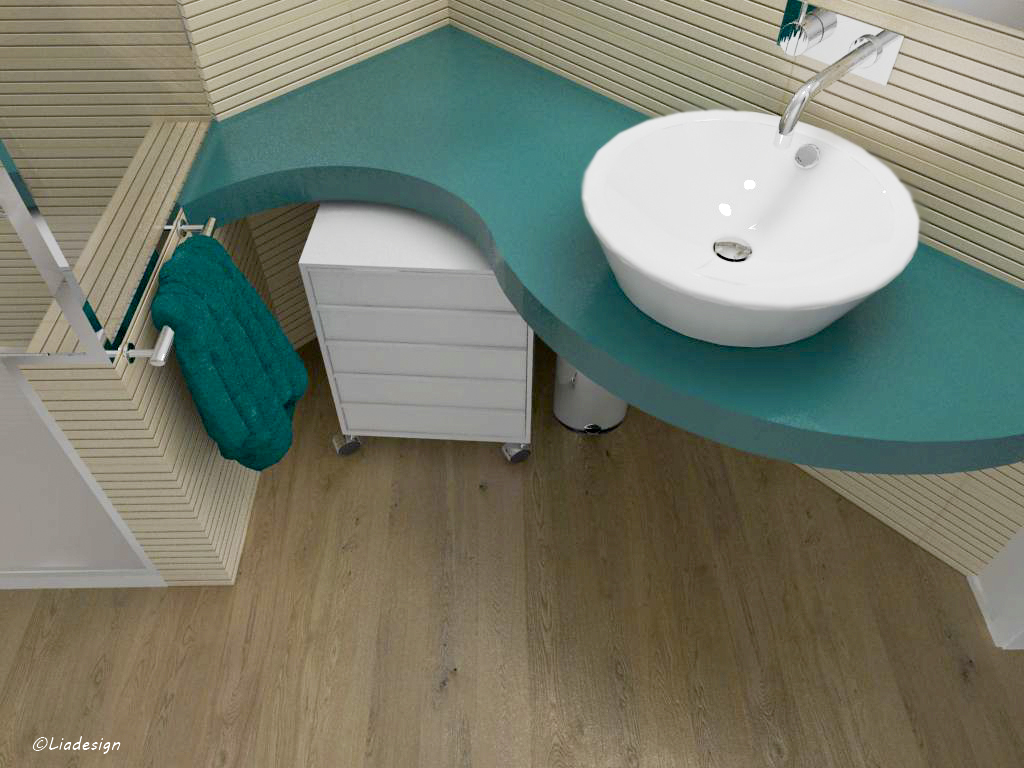The photograph depicts a modern bathroom characterized by horizontal wooden plank walls that give the space a sleek, rustic appearance. On the right-hand side of the image, the wooden wall serves as a backdrop for a dark green countertop that extends across the back of the room and curves to the right. A metal bar with a green towel, matching the countertop color, is attached to the front left portion of this wooden wall. Below the countertop, a white rolling cart with five handle-less drawers provides storage and sits on the light wood flooring that covers the ground. To the right of the countertop, there is a stylish, circular white sink resembling a large bowl. The sink is complemented by a long, skinny silver faucet protruding from the wall, with water currently flowing into the basin. A silver circular drain is located at the bottom of the sink, completing the functional yet sophisticated design of the bathroom.